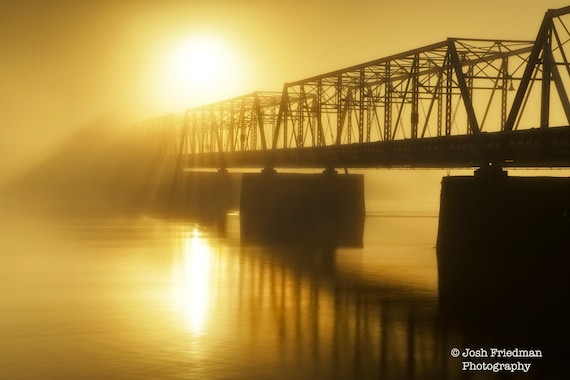A photograph captures an angled view of a steel girder bridge shrouded in fog during what appears to be sunrise. The bridge, with its triangular metal framework, stretches from the left side of the image, resting on three large rectangular concrete supports that plunge into the calm, reflective waters below. The hazy atmosphere and early-morning light cast a warm, golden glow over the entire scene, creating a brownish-orange, almost sepia-toned ambiance. The sun, centrally positioned above the bridge, enhances the ethereal quality, its light gently diffusing through the mist and reflecting off the serene surface of the water. The bridge, partially obscured by the fog, casts faint reflections in the tranquil waters, adding to the dreamlike quality of the photo. In the bottom right corner, the text "© Josh Friedman Photography" is prominently displayed in white font.